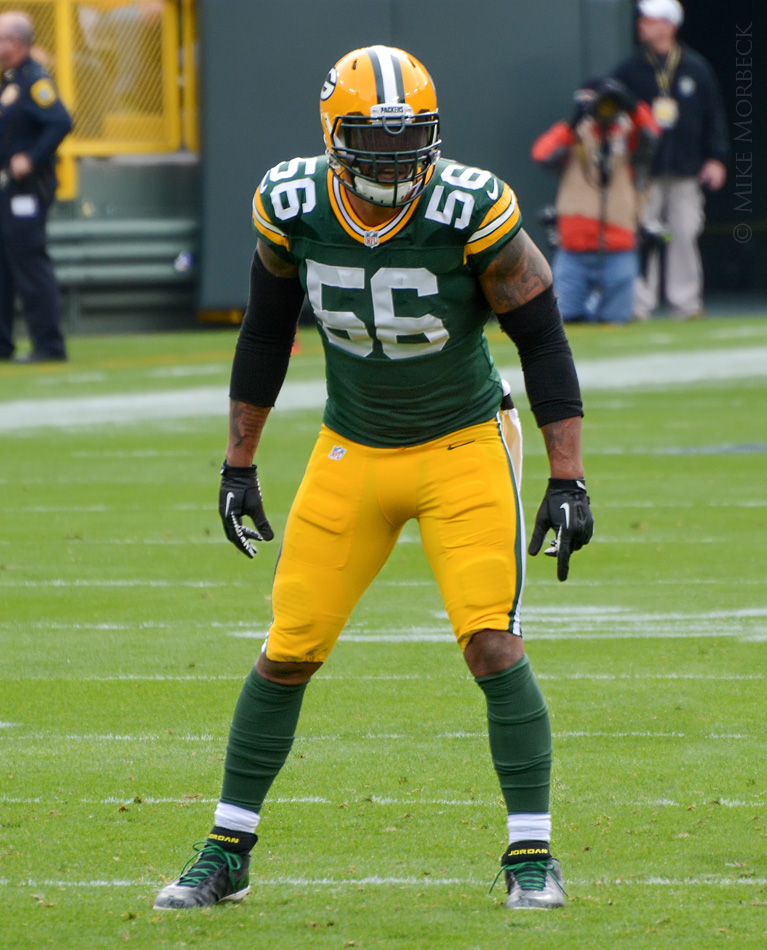The color photograph captures a moment during a Green Bay Packers football game, featuring a player, number 66, on defense, poised to tackle an opponent. The player, a black man with muscular arms adorned with tattoos, wears a distinctively green and yellow uniform. His ensemble includes a green jersey with white and yellow stripes, yellow pants with matching stripes, green shin protectors, white socks, and black shoes. His yellow helmet features a face guard, and he’s equipped with black Nike gloves. The green grass field is marked with white yard lines. In the background, several individuals, including a police officer, a photographer, and a stadium worker, stand blurred, emphasizing the player's intense concentration and readiness to pounce on his target.